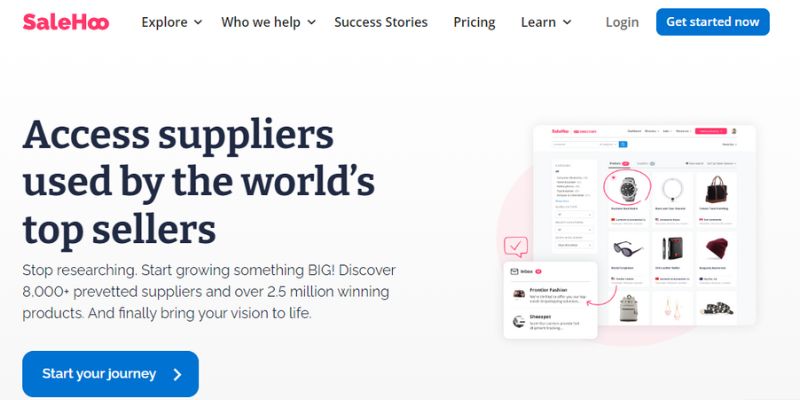The screenshot depicts a website interface for "SaleHoo," with its name prominently displayed in pink on the top left corner. The navigation bar spans the top and includes the following options: Explore, Who We Help, Success Stories, Pricing, Learn, Log In, and a blue "Get Started Now" button. The main page banner features a bold statement: "Access Suppliers Used by the World's Top Sellers," followed by a tagline encouraging visitors to "Stop Researching, Start Growing Something Big." It highlights the availability of over 8,000 pre-vetted suppliers and more than 2.5 million winning products, with a call to action button labeled "Start Your Journey."

On the right side of the main page, there appears to be a visual showcasing a variety of fashion items including a watch (which is circled), a necklace, a handbag, sunglasses, a hat, and potentially a backpack and earrings. An arrow from the sunglasses points to a side menu, the purpose of which is unclear due to the image quality.